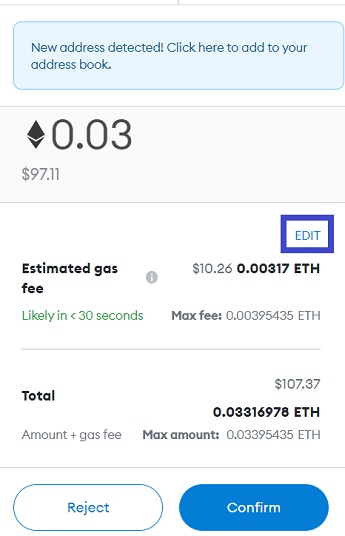A person is depicted on a checkout page where they're finalizing a purchase using Ethereum, a popular cryptocurrency. The interface features a notification in a light blue box that reads, "New address detected, click here to add to your address book." The payment section is clean and minimalistic with a white background. An area in the middle of the screen details the estimated gas fee, indicating the transaction cost for using Ethereum. At the bottom of the page, there are two primary action buttons: a blue "Confirm" button and a white "Reject" button. Additionally, a blue boxed outline highlights an "Edit" button, though its exact function remains unspecified in the image.